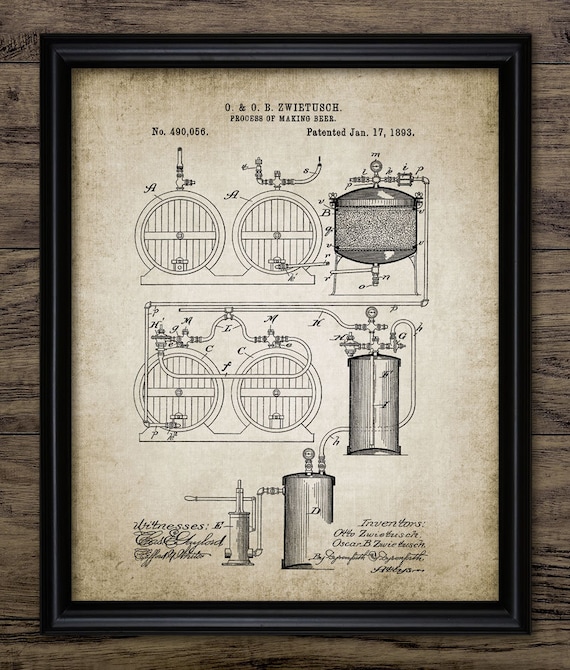The image showcases an artificially created photograph of a framed patent diagram on a dark brown wooden background, complete with wood grain detail. Enclosed in a sleek, black frame, the weathered parchment appears aged at the edges. The document, dated January 17, 1893, features a black-and-white schematic of a brewing system with multiple beer keg depictions, accompanied by technical text. At the top, it reads "O&O B. Zwietusch Process of Making Beer" and lists patent number 490-056. The detailed diagrams show various views and stages of the beer-making equipment, including cylindrical structures resembling kegs or silos with interconnected tubing. The bottom left holds hard-to-read classical print signatures marked “Witnesses,” while the bottom right lists the inventors: Otto Zwietusch, Oscar Zwietusch, and an unreadable third name in cursive.